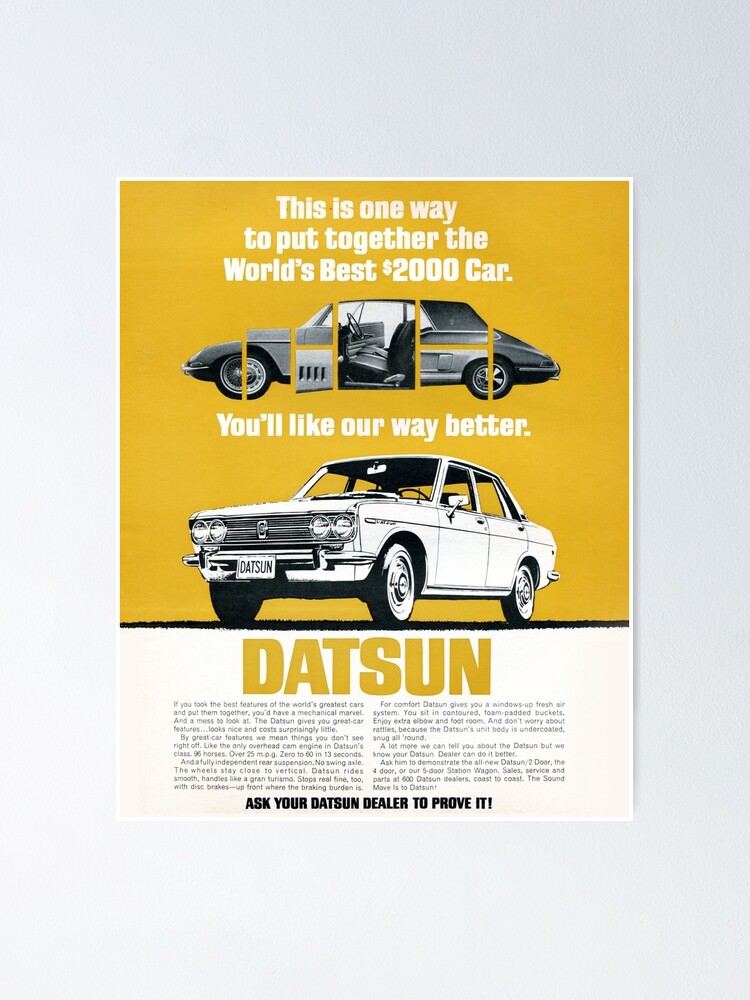This is an old magazine advertisement for Datsun, set against a striking orange background. The ad is notable for its playful and eye-catching design. At the top, bold text reads, "This is one way to put together the world's best $2,000 car," accompanied by an image that creatively pieces together mismatched segments of different cars. The assembly includes elements like a different hood, body, front, and back, altogether making up nine distinct sections to form a single, somewhat disjointed car. Below this, the text states, "You'll like our way better," leading into a three-quarter shot black-and-white line drawing of a complete Datsun, shown from wheel level looking up. Prominently displayed in bold orange letters is the word "Datsun," followed by smaller, nearly unreadable text and a final call to action: "Ask your Datsun dealer to prove it." The ad effectively contrasts the piecemeal car with a fully functional, sleek white Datsun, emphasizing the brand's superior construction.